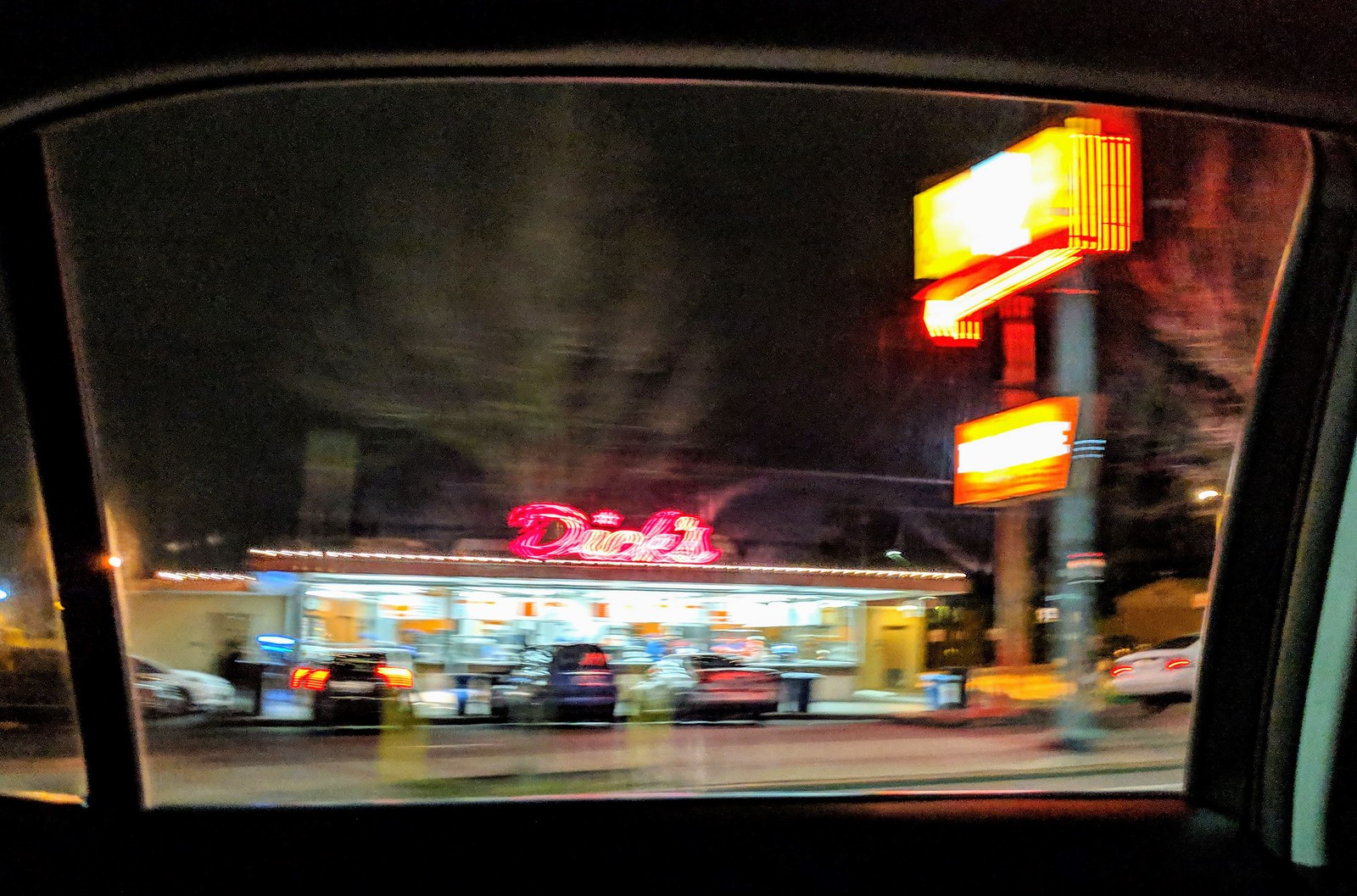A blurred photograph taken at night from the backseat of a moving car, framed in a rectangular shape with a car’s rear window in the foreground. The reflection of the person taking the photo is faintly visible in the bottom part of the window. Outside, against a dark night sky, sits a small, rectangular building with a large glass shop front. Atop the building, a red neon sign spells out "Dick's." The scene includes multiple cars parked in a small parking lot in front of the building. There's a prominent yellow sign lit brightly on two tall poles next to the building, casting a strong light but obscuring any readable text due to its brightness. A tree, large and vaguely discernible due to the blur, looms over the scene, completing the atmosphere of a bustling yet nighttime cityscape.